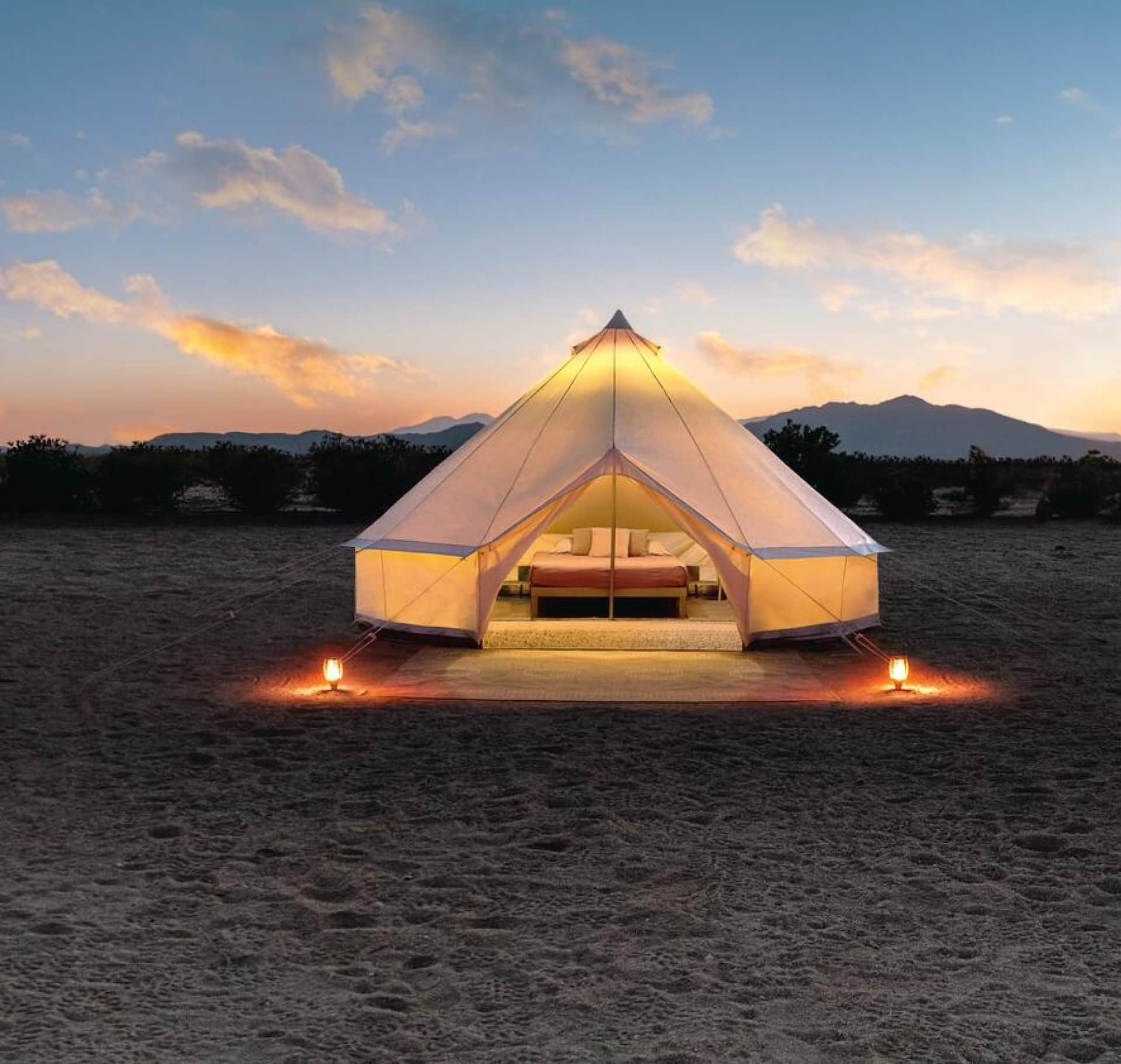The image is a color photograph in a square format, featuring a bell-shaped canvas tent situated on a sandy beach. This tent, centrally placed, boasts a large, white canvas exterior with a zip front door tied open by cables on both sides. It rests on a reddish-brown wooden platform, accented by a cream-colored rug at the entrance. Two lanterns, resembling candles, glow on either side of the deck, enhancing the ambiance. Inside the brightly lit tent, a bed draped in a brick-colored sheet and adorned with green and cream pillows is clearly visible, with a possible couch nearby. The footprints scattered across the sand around the tent add a touch of human presence, though no people are seen. A row of bushes and silhouetted trees lines the horizon, with mountains in the background. The sky above exhibits a beautiful post-sunset scene, with a blue gradient that fades into a pinkish-orange hue closer to the horizon, scattered with clouds. The overall atmosphere suggests a serene, luxurious camping (glamping) experience.